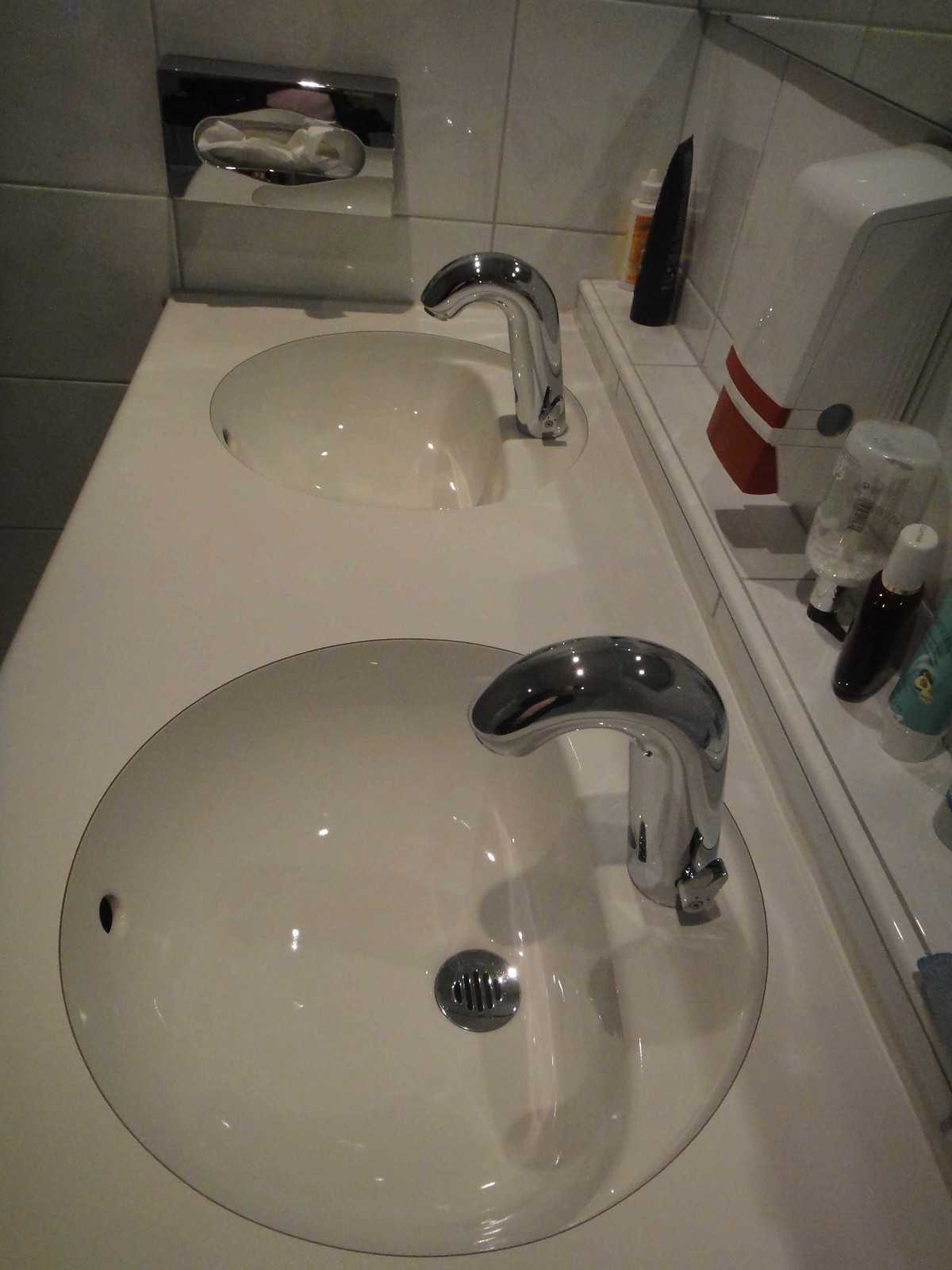The image depicts a bathroom with a double sink vanity featuring two circular white basins, each equipped with sleek silver faucets. The countertop is white and is mounted against a white rectangular tiled wall. The lighting is dim, creating a soft, low-light ambiance. Positioned between the sinks is a white soap dispenser marked with red or maroon buttons, typically activated by pushing the bottom part. Flanking this soap dispenser are several bottles, including a lotion bottle, a needle spray, and a squeeze-type lotion container. On the wall behind these items is a chrome tissue box dispenser with white tissues protruding from the top. Additionally, a glimpse of a rectangular mirror frame is visible at the upper part of the image, though the mirror itself is not fully shown. To the side, there is a public bathroom's silver paper towel dispenser. The overall setting gives a clean, organized, and slightly utilitarian feel typical of a public restroom.